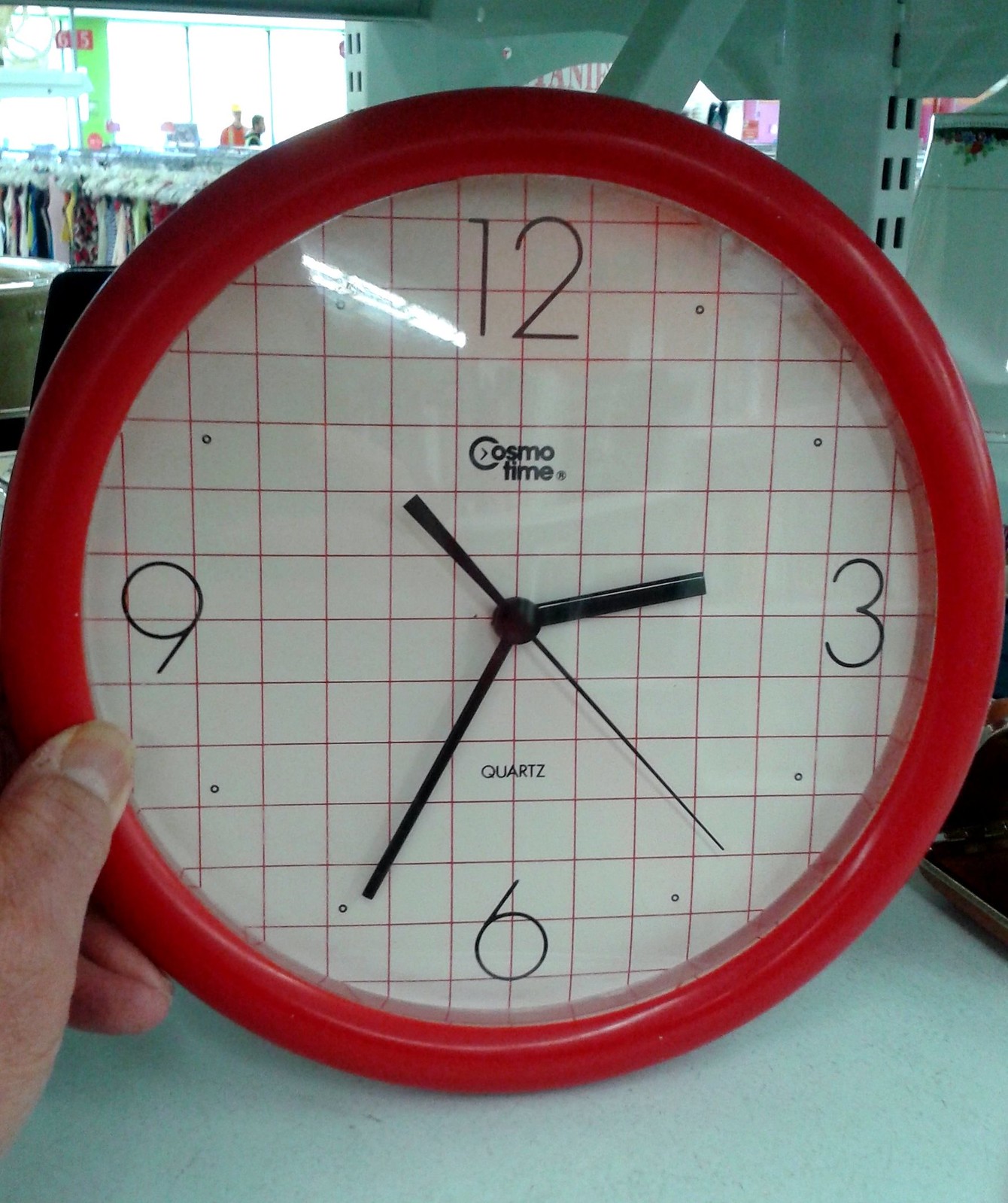In this detailed photograph taken inside a store, the upper left corner reveals the glass window front. Below the window, there is a rack displaying various women's dresses. Dominating the forefront of the image is an individual holding up a wall clock against a gray surface. The person’s thumb, which has a mid-range skin tone, is visible in the lower left corner and appears slightly unusual. The wall clock has a red plastic rim with a white face, featuring black striped squares marking the hours. Notably, only the numbers 12, 3, 6, and 9 are present. The clock has three hands for indicating the seconds, minutes, and hours.